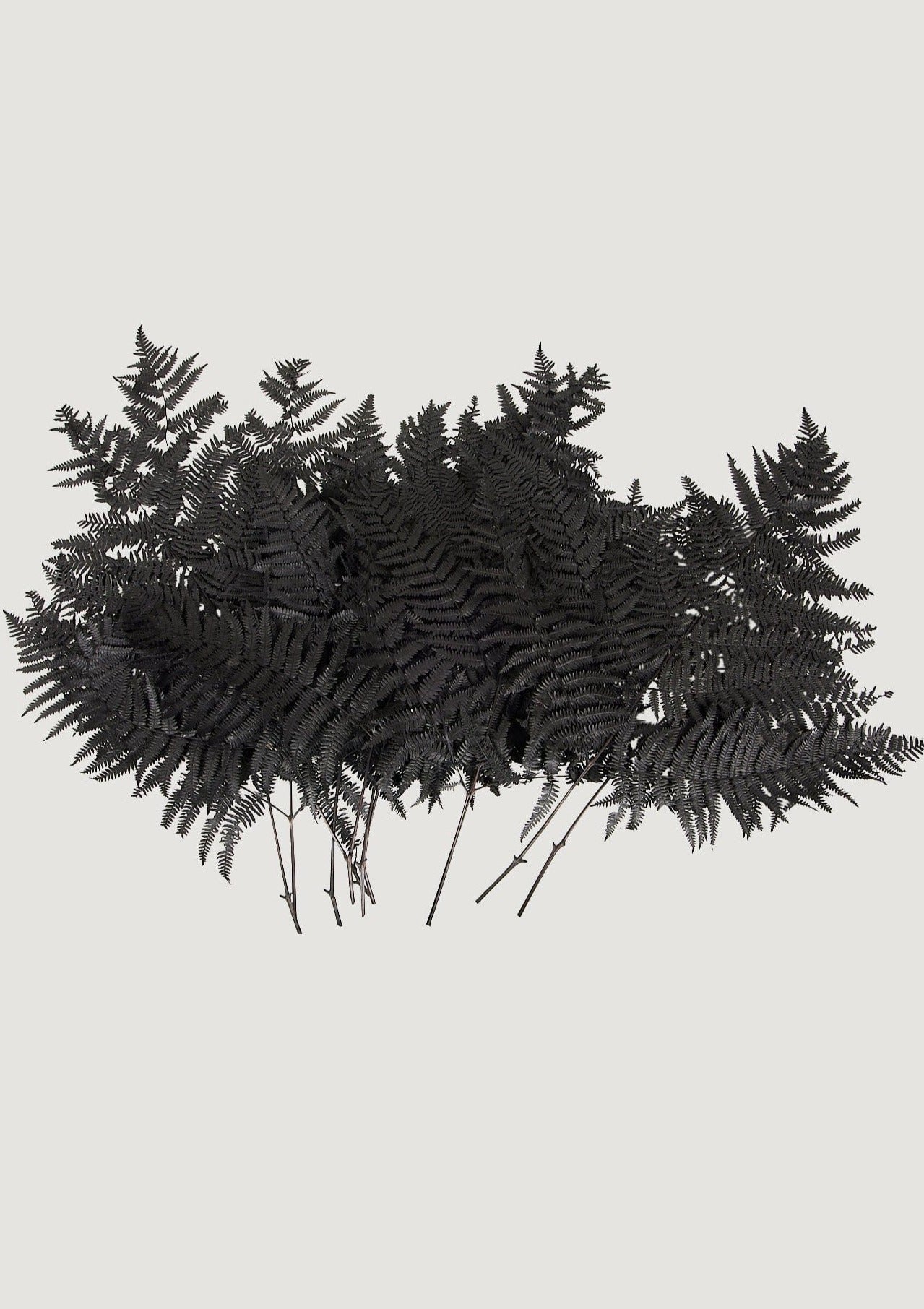A professional black-and-white photograph features a high-detail and textured display of fern leaves in the center, created likely through a special photographic process. The image has a completely white background at the top and bottom, with the ferns occupying the central space from left to right. These artistically aligned fern leaves are intricately detailed and appear almost like silhouettes against the varying tones of white to gray to black. The arrangement consists of multiple fern branches, their tips pointing upward and stems extending downward, creating a pattern that intersperses and fuses the leaves together. The fern branches exhibit a characteristic structure, with long, thin wooden strips for stems and leaves that decrease in size as they extend from the base to the tip. The scene evokes a sense of delicate yet vibrant design, accentuated by the ample white space above and below the central grouping of ferns.